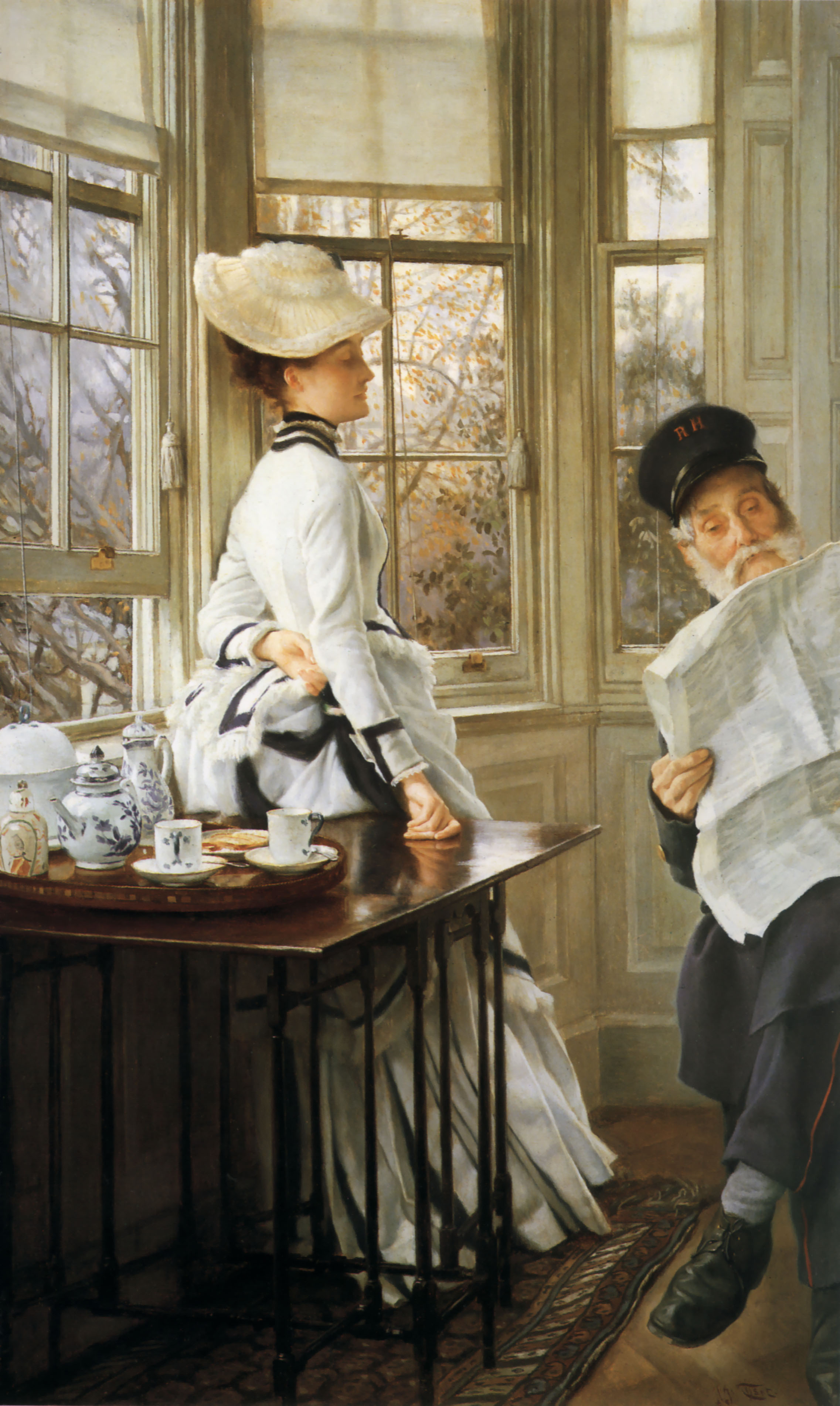This painting depicts a beautifully detailed interior scene from a bygone era, featuring a man and a woman in a room bathed in natural light from a partially open bay window with a view of leafy trees outside. The room boasts polished hardwood floors and a vibrant Victorian runner. 

On the left, a woman stands in a long, white, long-sleeved dress with black trim and a tan hat. She is leaning against an ornate, multi-legged side table adorned with an exquisite white tea set, which features blue patterns, including a tea kettle, two teacups with saucers, and other containers. Her right side profile is visible as she stands in front of the bay windows, with the furthest left window slightly ajar. 

On the right side of the painting, an elderly man is seated with his left leg crossed over his right, wearing a navy outfit, possibly a suit, black shoes, and gray socks. He is engrossed in reading a newspaper, which he holds up. A black hat sits atop his head, and his face is distinguished by a white beard and mustache. The composition captures a serene and genteel moment within a richly appointed room.